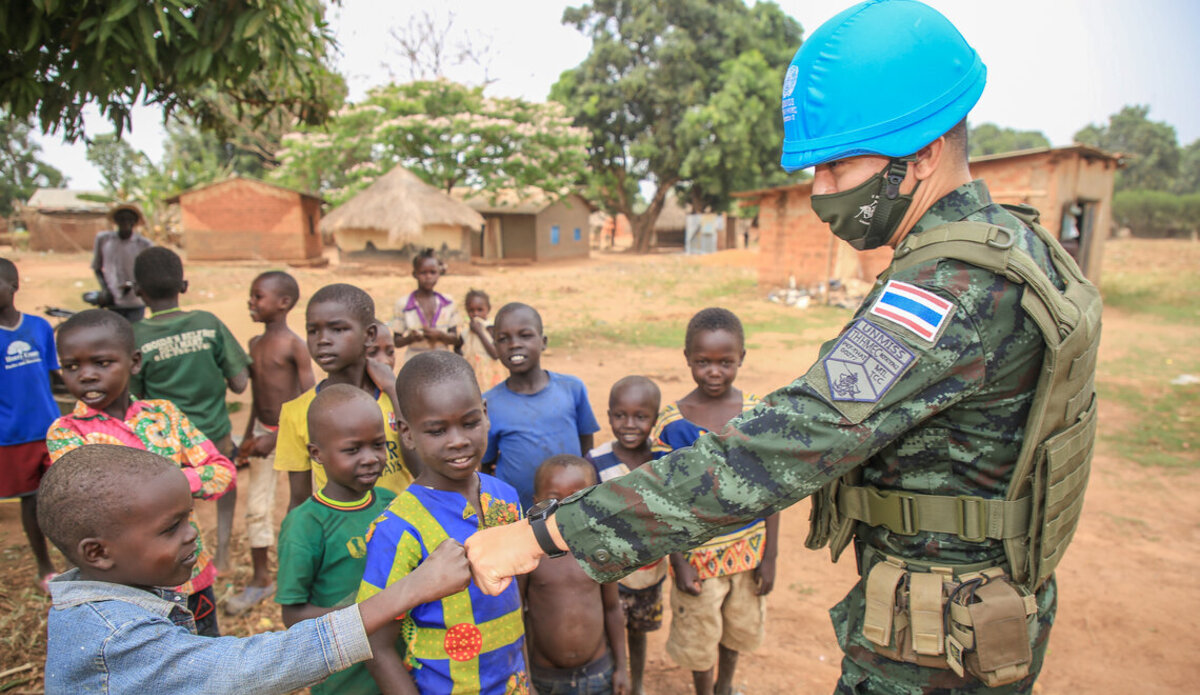In this outdoor photograph set in a small village, the focus is on a soldier with a light brown or olive complexion. He is dressed in green camouflage fatigues and an olive green tactical vest, adorned with tan pouches around his waist. His left sleeve features a patch with a flag marked by a blue stripe in the center, flanked by white stripes, and bordered by thin red stripes. He also wears an army green face mask and a distinctive bright light blue helmet. The soldier's left arm is extended in a fist bump with a small African American boy sporting a jean jacket. Surrounding them is a group of African American children, some smiling, others watching intently, and a few shirtless, all gathered on a sandy, sparsely grassed lot. The background reveals several small huts, constructed out of wood and mud, with one appearing to be made of brick. Trees are scattered among the huts under a clear blue sky, devoid of clouds.